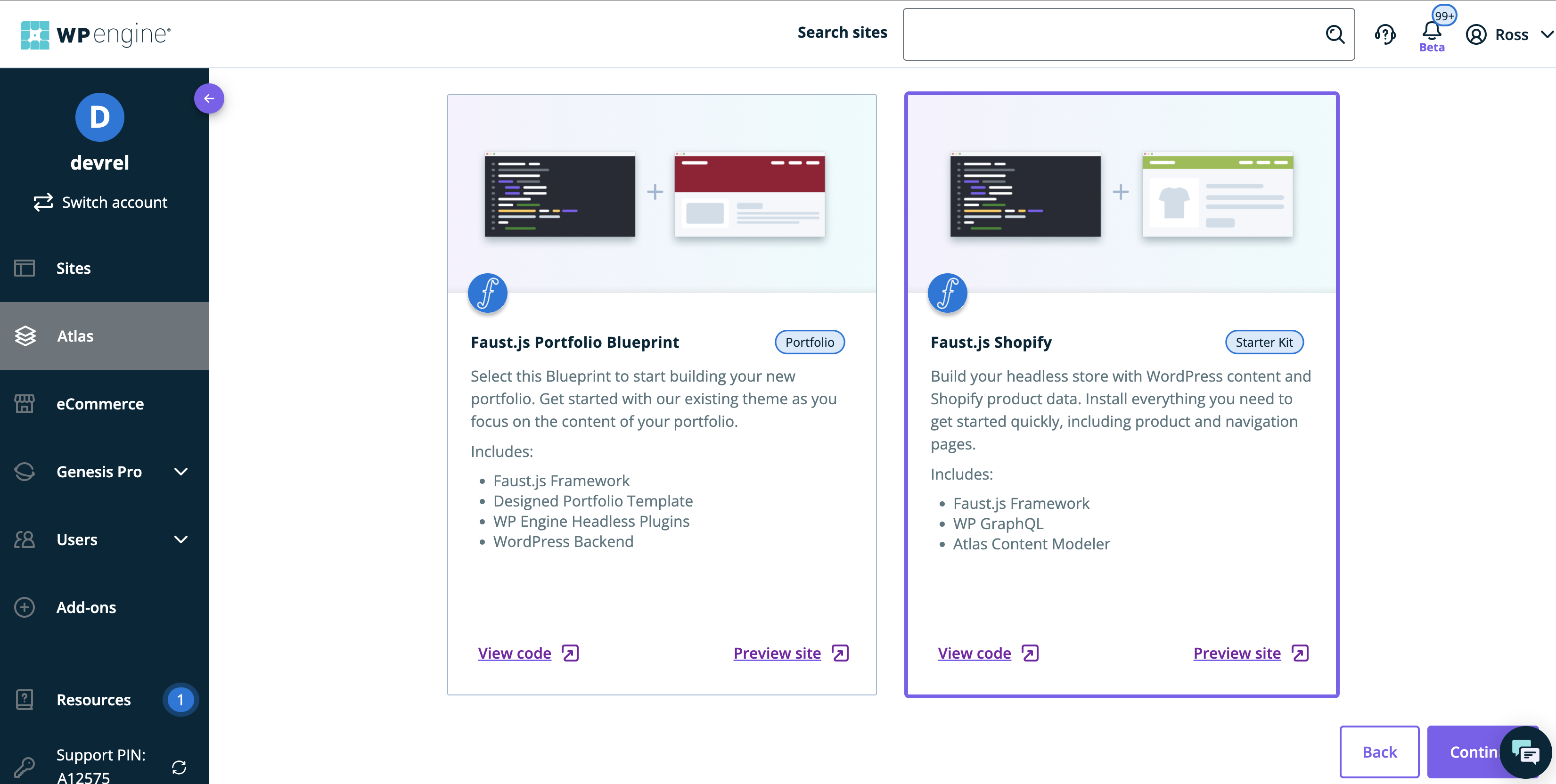The image is a screenshot of a website with a predominantly white background. In the upper left corner, the bold text "WP Engine" is prominently displayed. Adjacent to this, there is a logo featuring a light blue box with white accents. Towards the right side, there is a "Search site" label next to a search bar. 

In the upper right corner, a notification bell icon is visible, displaying "99+" notifications with the word "Beta" beneath it. Next to the bell, the name "Ross" is displayed.

On the left side of the image, there is a vertical navigation bar. At the top of this bar, there's a blue circle with a white "D" in the center and the label "DevRel" beneath it. Below this, the navigation options are listed as follows: "Switch Account," "Sites," "Atlas," "E-commerce," "Genesis Pro," "Users," "Add-ons," and "Resources." The "Resources" option is highlighted with a blue circle containing the number "1" beside it. Further down, there is an option labeled "Support" next to which is a pin icon. Below "Support," there is a key icon with the text "A12575" next to it.